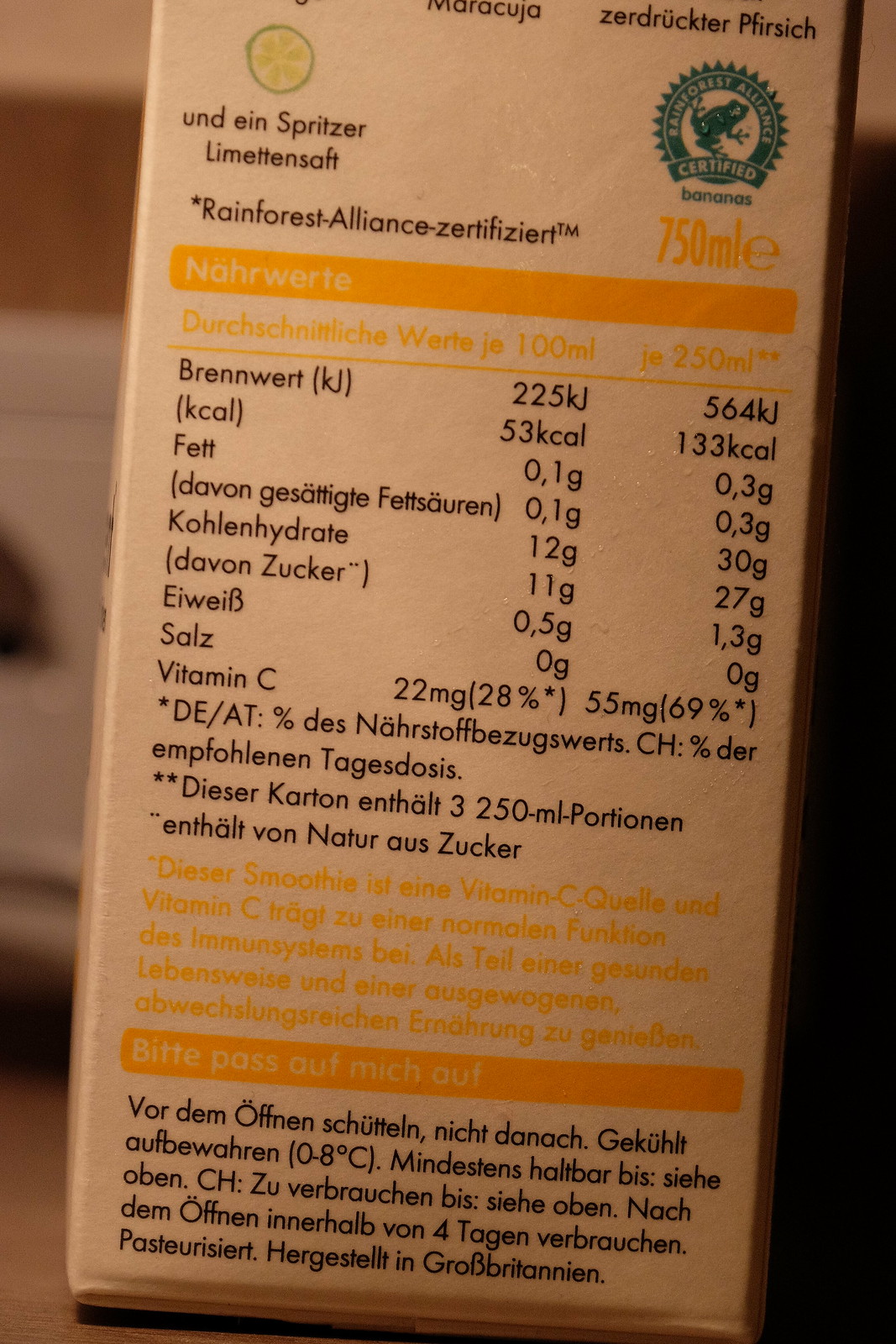This detailed close-up photograph captures the back of a primarily white cardboard carton, likely for a beverage such as milk or orange juice. Prominently, there is a graphic of a lime cut in half, revealing a lighter green interior with a spiral-like pattern, situated at the top left-hand side. The text on the carton is predominantly in German, with a conspicuous focus on health or nutritional information. Among the text, the word "smoothie" is highlighted in yellow. Additionally, an identifiable emblem appears on the right-hand side: a dark green circle accented with triangular shapes around the perimeter, featuring a silhouette of a frog in the center. Under this frog, a ribbon-like banner inscribed with the word "certified" spans across, while the phrase "Rainforest Alliance Certified" encircles the frog. The term "bananas" is also noted beneath this emblem. The emblem signifies that the product meets certain sustainability standards.